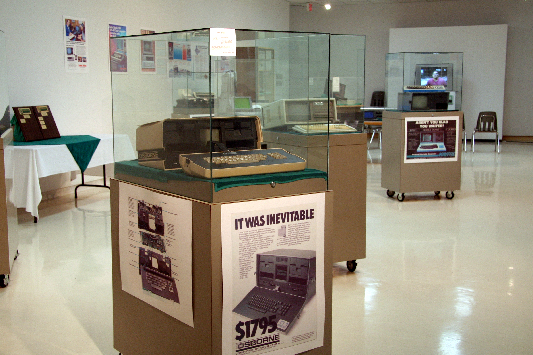The photograph showcases an indoor scene of a computer and electronics museum, focusing on a series of display cases that house early computer terminals, likely from the 1950s or 60s. Each display consists of a rectangular cardboard-like pedestal topped with a lucite or glass cube, encasing the antique computers. The computer monitors resemble oscilloscopes turned on their sides, and each pedestal has an advertisement poster affixed to it, one of which reads "It was inevitable," with a price of $1,795.

In the immediate foreground, slightly left of center, stands a large computer with a substantial keyboard, encased in its glass display. To its right and in the far background are additional display cases, each showcasing different early computer models. The setting features a white linoleum floor reflecting the fluorescent lights above, enhancing the sterile, archival atmosphere of the museum.

On the left side of the image, a series of posters are affixed to the white wall, running the length of the room. There is also a white banquet table adorned with a green banner and what appears to be a poster or plaque positioned atop it. In the far end of the photograph, a large whiteboard on wheels is visible, in front of which stands a smaller table surrounded by multiple chairs, adding to the educational and informative ambiance of the museum display.